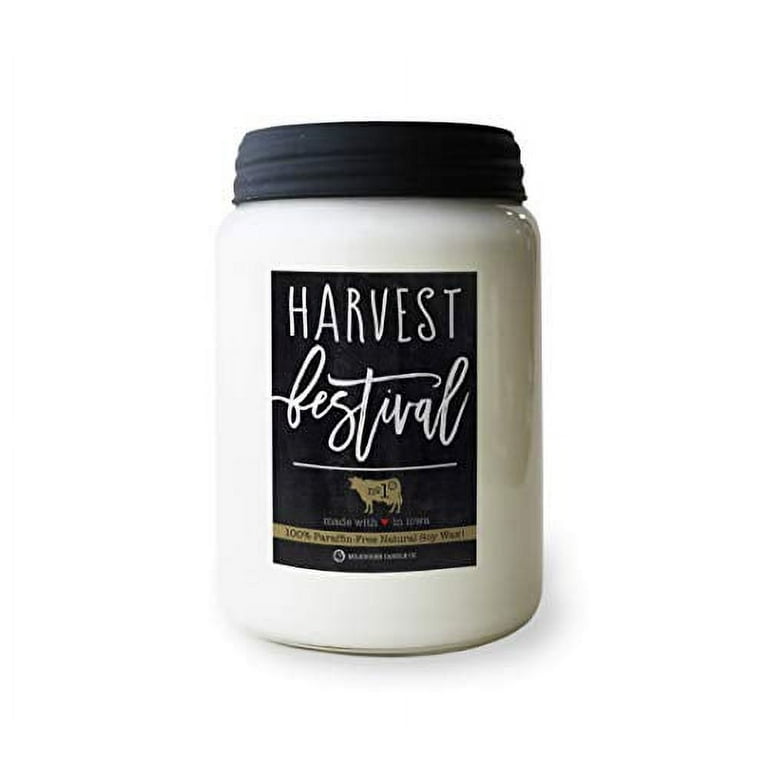This image is a product advertisement featuring a white glass jar with a black screw-on lid, standing against a white background. The jar contains a white substance. The label on the jar is black with white text, prominently displaying the product name "HARVEST" in all caps and "Festival" in cursive below it. The label also features a gold emblem of a cow with the text "number one" inside the image. Additional label details include the phrases "100% paraffin-free natural soy wax" and "made with love in town." The jar and its detailed labeling suggest it contains a high-quality, natural product, potentially a candle, given its soy wax content.